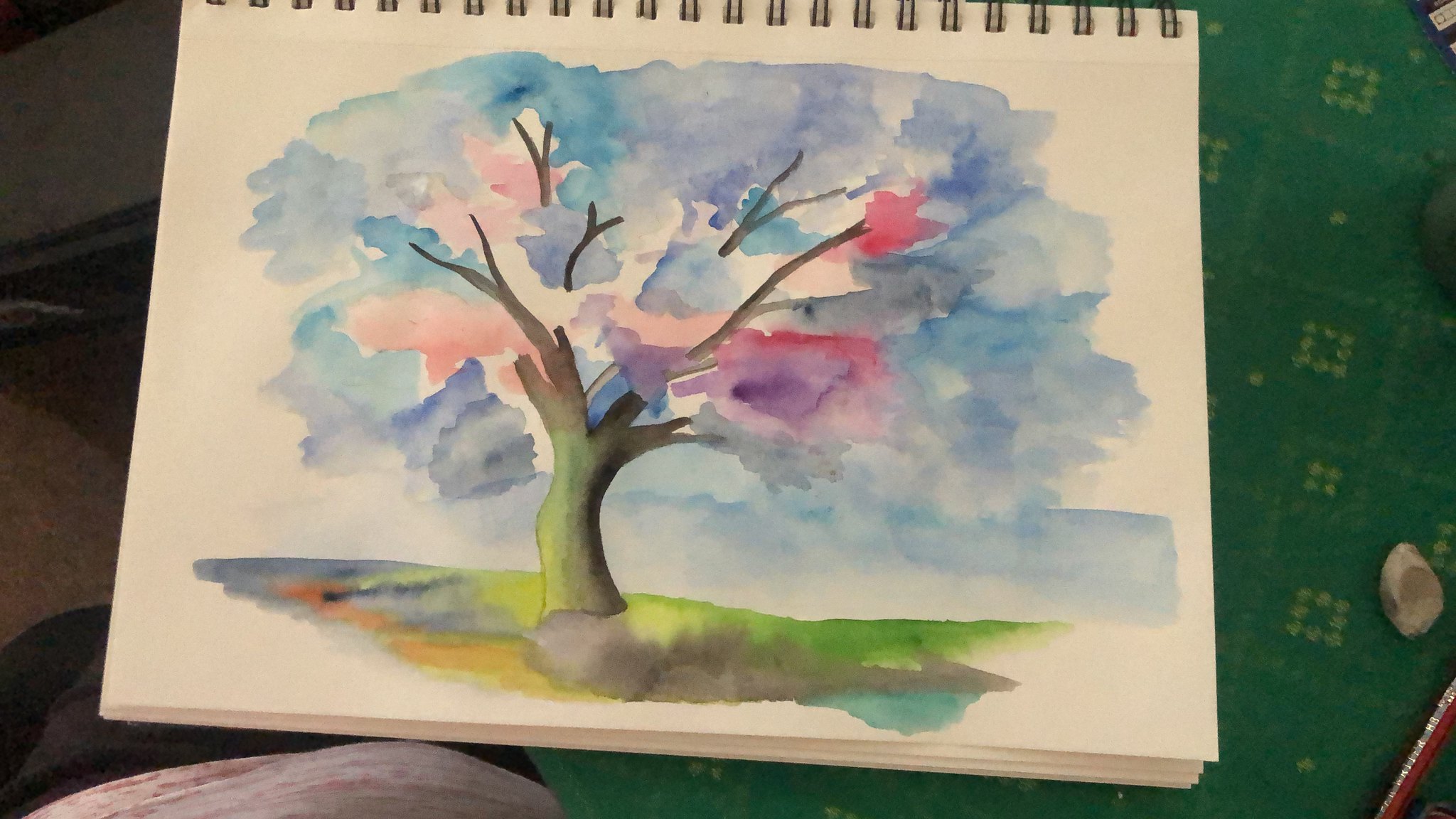This detailed image captures a spiral-bound art notebook with an off-white, slightly muted page on which a watercolor painting is depicted. The painting features a large tree with a trunk that transitions smoothly from light green to brown, and branches that stretch upwards. The leaves of the tree are rendered in a harmonious blend of blues, pinks, and purples with some subtle black accents, creating a vibrant yet soothing canopy. The ground below the tree is a textured mix of greens, yellows, grays, and hints of orange and black, suggestive of grassy areas and rocks, with no rigid boundaries between the colors. Notably, the scene includes a band of blue at the base, indicative of a body of water or sky. Adjacent to the notebook, the background features a green fabric with a pattern of lighter green squares formed by dots. Accompanying the notebook are an eraser, positioned on either the bottom left or right, and a red pencil. The entire artwork is free of outlines, emphasizing the fluid and blended nature of the watercolor medium.